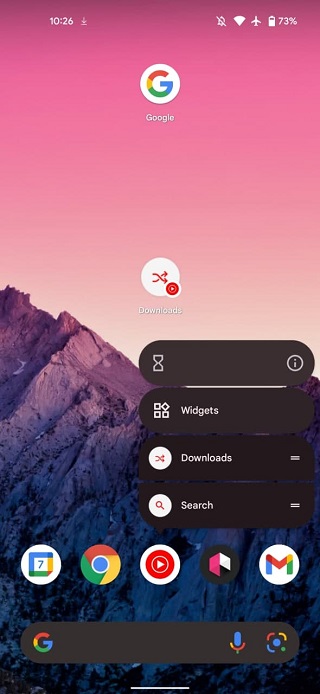The screenshot captures a breathtaking nature scene centered around a mountain ridge that spans the background. The sky above is a brilliant display, transitioning seamlessly from hues of magenta to soft whites, forming a stunning gradient. The mountain range below mirrors this colorful spectacle, displaying a spectrum of colors that flow from vibrant pinks and purples to deep blues and blacks, creating a mesmerizing, almost surreal landscape.

This spectacular image is viewed within a mobile phone interface, specifically captured from a Google application, as indicated by the round Google logo positioned at the top of the screen. The title "Google" is clearly present above the logo. Just beneath the logo is an icon representing downloads. Below this section, a series of stacked windows are displayed, featuring icons for widgets, another for downloads, and a prominent search window.

Towards the bottom of the screen, there is a horizontal row of five icons, with one prominently displaying the Google Chrome logo. Directly below this row, there is a dark gray search bar adorned with the Google logo at the beginning, completing the layout of the screenshot. The image blends technological elements seamlessly with the natural beauty of the mountain scene, creating a captivating visual experience.